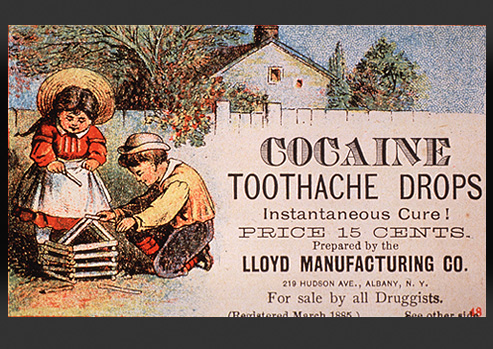This is an old advertisement from March 1885 for "Cocaine Toothache Drops" with an instant cure claim, priced at 15 cents. Prepared by the Lloyd Manufacturing Company, 219 Hudson Avenue, Albany, New York, and available for sale by all druggists. The ad features a colorful, cartoon-like illustration set within a wide vertical rectangular image bordered with a gray trim. The scene depicts two children with rounded faces playing outside. The girl on the left stands wearing a colonial-style red dress with a white apron and knee-length white socks, topped with a large straw hat. The boy is kneeling beside her, dressed in a small hat, a long-sleeved yellow shirt, and black pants. They appear to be constructing a house out of sticks, reminiscent of Lincoln logs. Behind them, there is a wooden plank fence, green trees, and a two-story house against a backdrop of a blue sky.